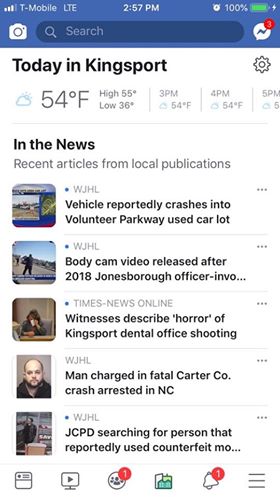This screenshot, taken from a mobile phone interface, captures a detailed view of various app interactions and notifications. The background at the top is a medium blue with three out of four signal bars, T-Mobile LTE service, the current time at 2:57 PM, an alarm icon, and a fully charged battery at 100%, indicated by a green battery icon with a lightning bolt suggesting it is charging.

Below the status bar, there is a section twice its height, featuring a generic camera icon on the left, a central search bar with a magnifying glass icon, and what appears to be the Messenger app with three notifications indicated by a red bubble and white text over a lightning bolt icon in a white speech bubble.

The subsequent section has a white background and black text. It presents a weather report for Kingsport, indicating partly cloudy conditions with a light blue cloud icon, a current temperature of 54°F, high of 55°F, and low of 36°F. The forecast details follow for 3 PM and 4 PM, both at 54°F, before being cut off.

Further down, the interface displays five recent news articles, predominantly from WJHL and one from Times News Online, all concerning law enforcement topics. Each article has a small thumbnail image, publication source, and brief headlines such as:
1. "Vehicle reported crashes into volunteer park where used car lot"
2. "Body cam video released after 2018 Jonesboro officer"
3. "Witnesses describe horror of Kingsport dental office shooting"
4. "Man charged in fatal car company crash arrested in North Carolina"
5. "JCPD searching for person reportedly using counterfeit currency," which appears cut off at the end.

At the bottom, a row of six icons against a white background includes:
1. A credential-like icon resembling a square divided in half with a dot and lines in the top part.
2. A play button within a TV-shaped icon.
3. A group of humanoid shapes within a circle, accompanied by a red notification bubble with the number one.
4. A factory-like icon in green and white.
5. A bell icon representing notifications with a red bubble and the number one.
6. A three-stripe hamburger menu icon.